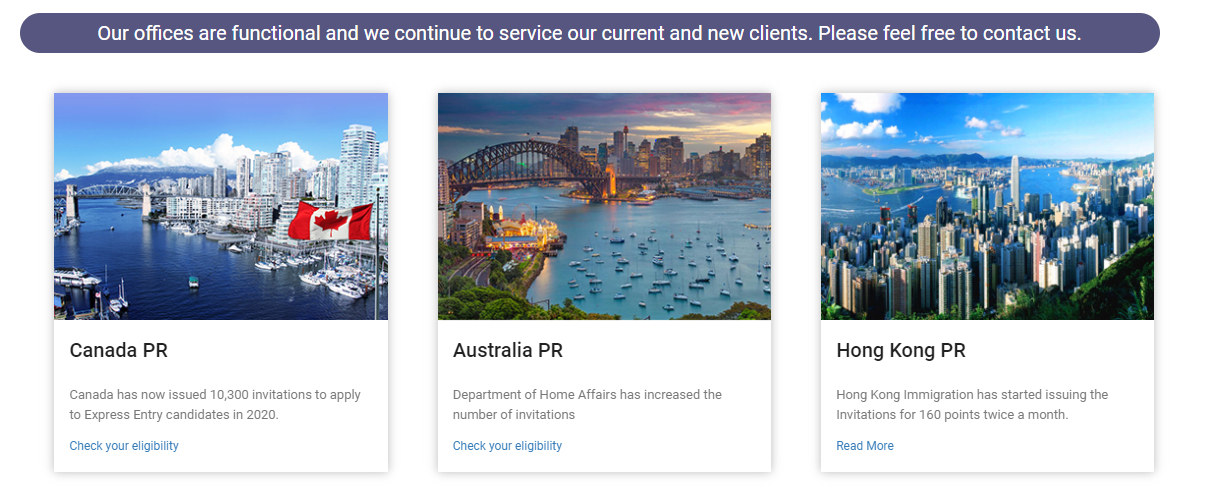**Web Page Overview: Travel Destinations Highlighting Canada, Australia, and Hong Kong**

**Top Section:**
- The web page has a clean white background. At the top, there is a prominent purple oval bezel with bold white text reading: "Our offices are functional, and we continue to service our current and new clients. Please feel free to contact us."

**Canada Section:**
- A beautiful depiction of Canada's shoreline features numerous gray and white buildings alongside white ships dotting the dark blue waters. 
- In the background, a majestic dark blue mountain is partially hidden by cascading white clouds, all set against a dark blue sky tinged with cyan hues. 
- The scene includes a blue and gray drawbridge supported by two large white pillars.
- Text under the image reads:
  - **Canada PR** (in bold black)
  - "Canada has now issued 10,300 invitations to apply to Express Entry candidates in 2020."
  - A hyperlink in blue text urges readers to **"check your eligibility."**

**Australia Section:**
- This section showcases Australia's landscape, featuring a large drawbridge amid numerous ships and buildings.
- The sky is an enchanting mix of gray, purple, violet, red, and blue tones.
- Text accompanying the image reads:
  - **Australia PR** (in bold black)
  - "Department of Home Affairs has increased the number of invitations."
  - A blue hyperlink invites users to **"check your eligibility."**

**Hong Kong Section:**
- Hong Kong's dynamic cityscape is presented with buildings in gray, light gray, tan, and red hues set against a dark blue body of water and a cyan blue sky with dark blue and white clouds.
- On the horizon, a city with more gray and tan buildings is visible.
- Text beneath the image includes:
  - **Hong Kong PR** (in bold black)
  - "Hong Kong Immigration has started issuing invitations for 160 points twice a month."
  - A blue hyperlink suggests readers to **"read more."**